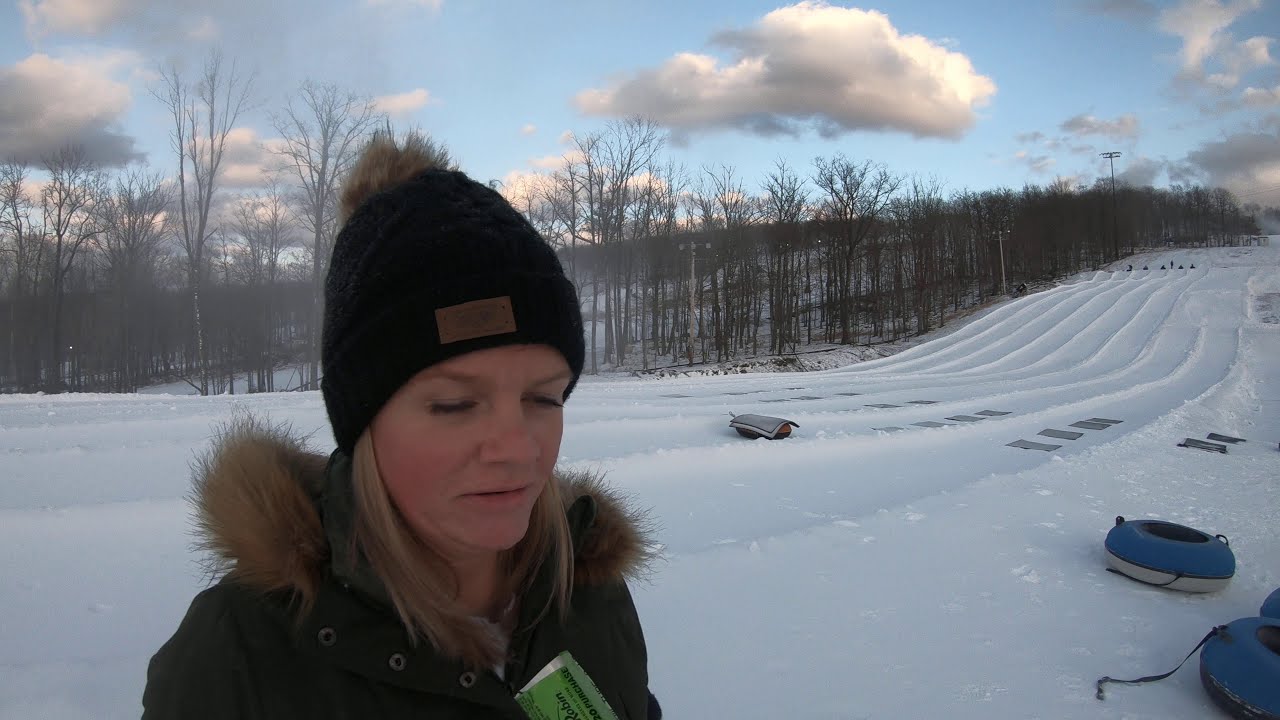In the image, a young woman stands on the left side in a snowy field, where snow tubing activities are underway. She has shoulder-length, blonde hair and is wearing a brown coat with a furry hood. On her head, she dons a brown knit hat, and she's looking downwards. To her right, there's a snow tubing course defined by several lanes, with blue inner tubes—one fully visible and parts of two others—stacked on that side. In the background, you can see the heads of other people near the tubing course. Further beyond, a snow-covered field stretches out, bordered by a line of trees. The sky above the trees features a large cloud and a few smaller ones scattered across it, suggesting a crisp winter day at a snow-covered resort.